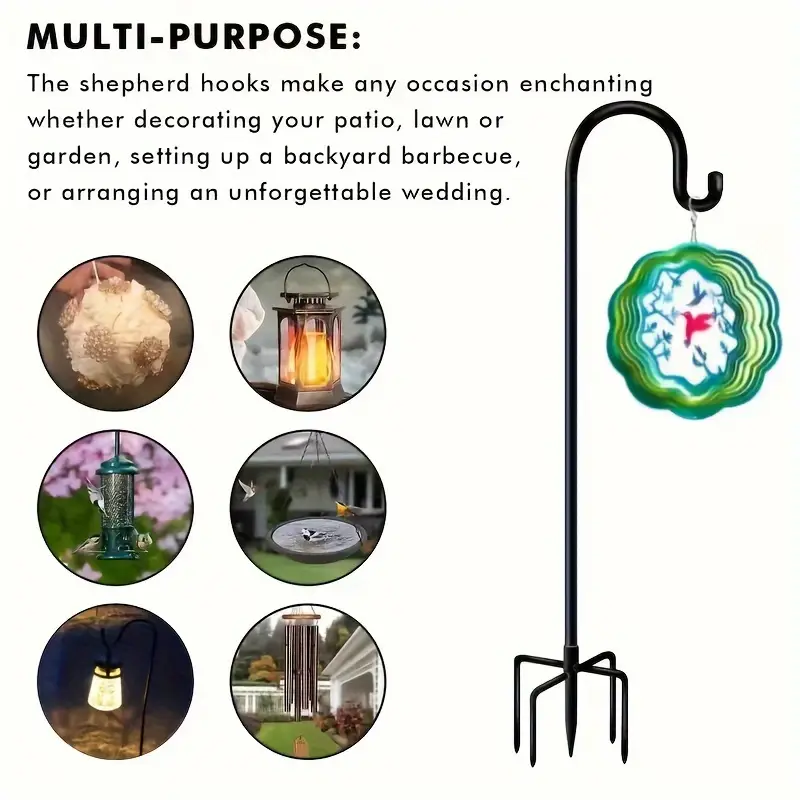This advertisement for shepherd hooks features a detailed layout against a pale peach-pink backdrop and is described as a square image approximately six inches in height and width. At the top-left corner, bold black text reads "Multi-purpose:" followed by four lines explaining that the shepherd hooks can make any occasion enchanting, whether decorating a patio, lawn, or garden, setting up a backyard barbecue, or arranging an unforgettable wedding.

On the right side of the image is a prominent illustration of the black metal shepherd's hook. This hook has a main pole supported by an innovative five-point base, featuring one central spike and four additional spikes forming an X-shape for enhanced stability. The pole extends upwards, curving into a crook at the top, ending in a loop. The loop holds a sun catcher with a red hummingbird and decorative spirals in green and blue.

To the left of the pole, there are three rows of circular insets arranged in two columns, illustrating various uses for the shepherd hook. The upper left circle features a Christmas ornament or bauble, while the upper right displays a lantern. The center row shows a bird feeder on the left and a bird bath on the right. In the bottom row, the left circle exhibits a nightlight, and the right one presents wind chimes. This arrangement highlights the versatility and multi-purpose nature of the shepherd hooks, making them suitable for a wide array of decorative and functional applications.